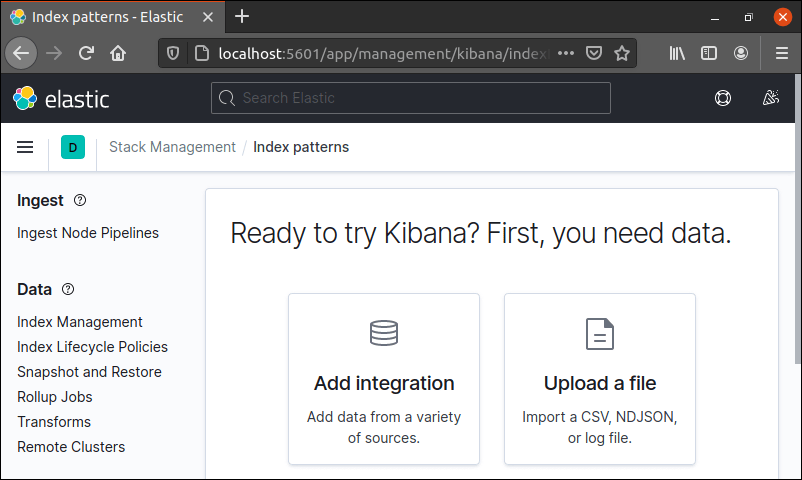The image features a light blue background with a black top section. At the top, there are clusters of small circles in blue, green, red, and yellow. Text reading "Index Patterns / Elastic" is displayed, accompanied by an 'X'. Below this, a large search box is situated, ending with a red circle containing an 'X'. To the left of the search box, a highlighted left arrow appears, followed by a right arrow, a backup icon, and a house icon. Another search box below references 'localhost', 'management', and 'Kibana', and is flanked by various icons, including three lines.

Further down, there's an elastic logo with several colorful balls and another search box. Nearby, a small circle encloses a square, and an icon resembling a fallen tree is present. 

On the white section, a white box contains three black lines, a green box with a 'D', and text that reads "Stack Management Index Patterns". Against the blue background, the word "Ingest" appears with a circle containing a question mark, followed by "Ingest Node Pipelines". Further labels include "Data", another question mark inside a circle, "Index Management", "Index Lifecycle Policies", "Snapshot and Restore", "Rollup Jobs", "Transforms", and "Remove Clusters".

A prominent white box in the center prompts users with, "Ready to Try Kibana? First You Need Data". It offers two options: "Add Integration" and "Add Data from a Variety of Sources". Below these, instructions are given to "Upload a File" and "Import a CSV, JSON, or Log File". Lastly, there is a grey slide button on the right.